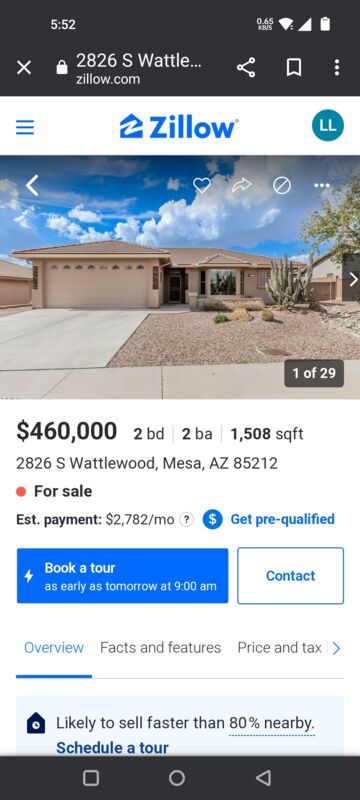This is a detailed caption for the image provided:

The image is a screenshot of the Zillow.com website displayed on a mobile device. At the top of the page, the recognizable Zillow logo is prominently featured, showcasing a blue house icon with a white "Z" centered within it. Below the logo, the main listing appears, displaying a property located in Mesa, Arizona. The home is a beige-brown color and is surrounded by a desert landscape that includes cacti plants and small stones or pebbles. The property listing indicates that there are a total of 29 images available for viewing, with the option to swipe through them. The home is listed for $460,000 and features two bedrooms, two bathrooms, and offers 1,500 square feet of living space. Below the property details, there is a button allowing users to book a tour or contact the listing agent.